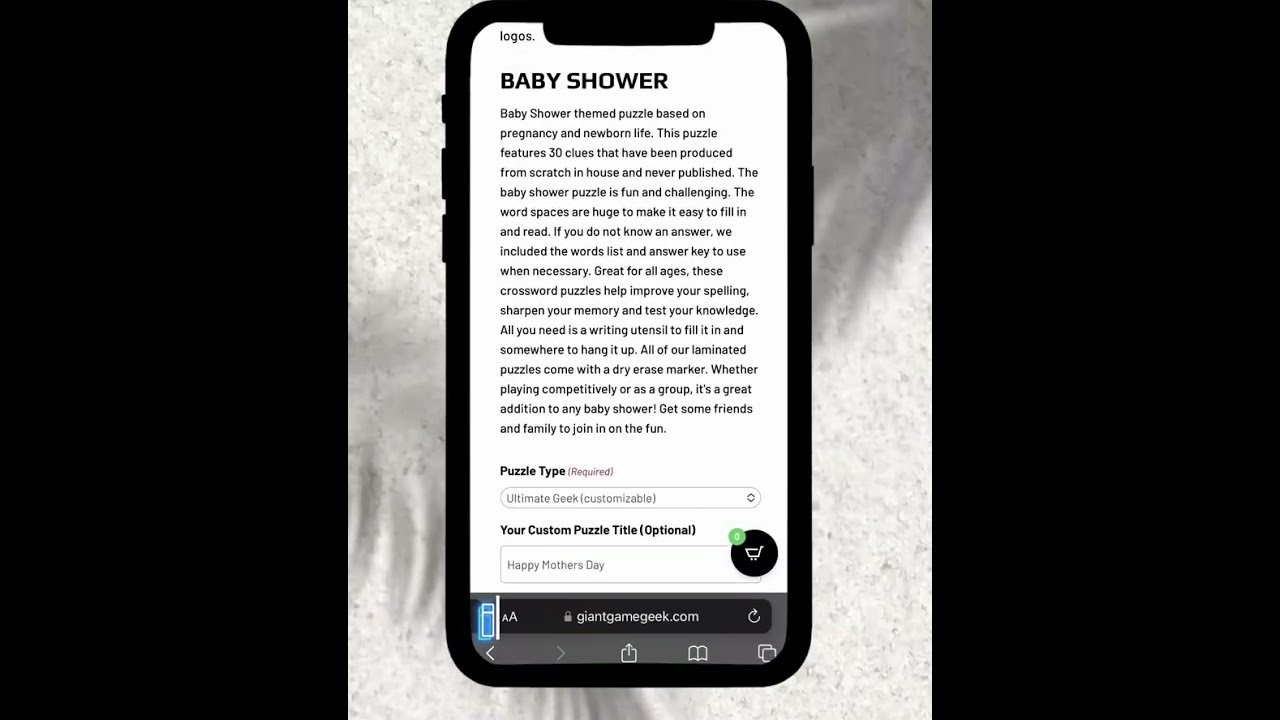In the image, a smartphone is displayed on a tabletop, surrounded by black bars on the left and right edges. The phone’s screen is white, featuring a webpage from giantgamegeek.com, which showcases a customizable baby shower-themed puzzle. At the top-left of the screen, the word "logos" is visible. Below it, in bold black capital letters, it reads "BABY SHOWER." The description underneath provides details about the puzzle, stating "Baby shower themed puzzle based on pregnancy and newborn life. This puzzle features 30 clues that have been produced from scratch in-house and never published. The baby shower puzzle is fun and challenging. The word spaces are huge to make it easy to fill in and read. If you do not know an answer, we include the word list and answer key to use when necessary. Great for all ages, these crossword puzzles help improve your spelling, sharpen your memory, and test your knowledge. All you need is a writing utensil to fill it in and somewhere to hang it up. All of our laminated puzzles come with a dry erase marker. Whether playing competitively or as a group, it's a great addition to any baby shower!" Beneath this description is a section labeled "Puzzle Type" with a customizable option box, and a selectable "Ultimate Geek Customizable" box. Below this, there's text that reads "Your custom puzzle title (optional). Happy Mother's Day." Adjacent to this is a shopping cart icon and a black box with a refresh sign. The image captures the essence of ordering a personalized, enjoyable puzzle for a baby shower, reflecting the engaging and thoughtful nature of the gift.